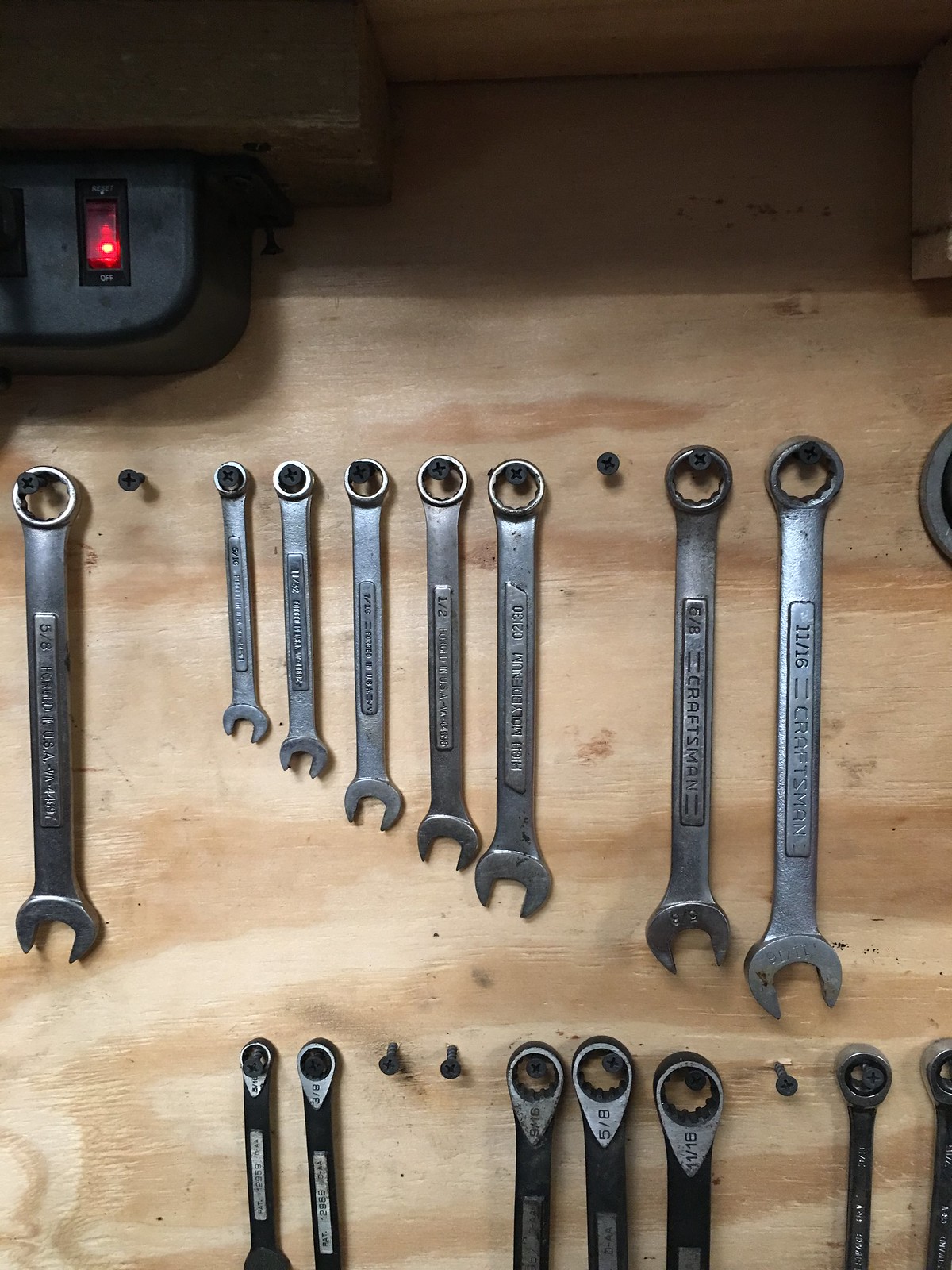The image displays a meticulously arranged set of tools, primarily wrenches, organized on a wooden board mounted on a wall. There are a total of seven metallic silver wrenches hanging prominently from screws arranged in ascending order of size from left to right, except for one larger wrench located on the far left. Below them, another set of seven similar wrenches in black color partially obscured from view. The screws and nails, some empty, are evenly spaced and support the tools. 

Detailing further, these tools are inscribed with sizes such as 11, 16, 6, 8, 1, and 2, including a wrench labeled with 6/8 on the left. Above the wrenches on the right side, the brand name "Craftsman" is visible. Additionally, in the top left corner is a black object mounted upside down with a label indicating "off" and a red-lit switch, affixed to the wooden board within this organized cabinet-like space.